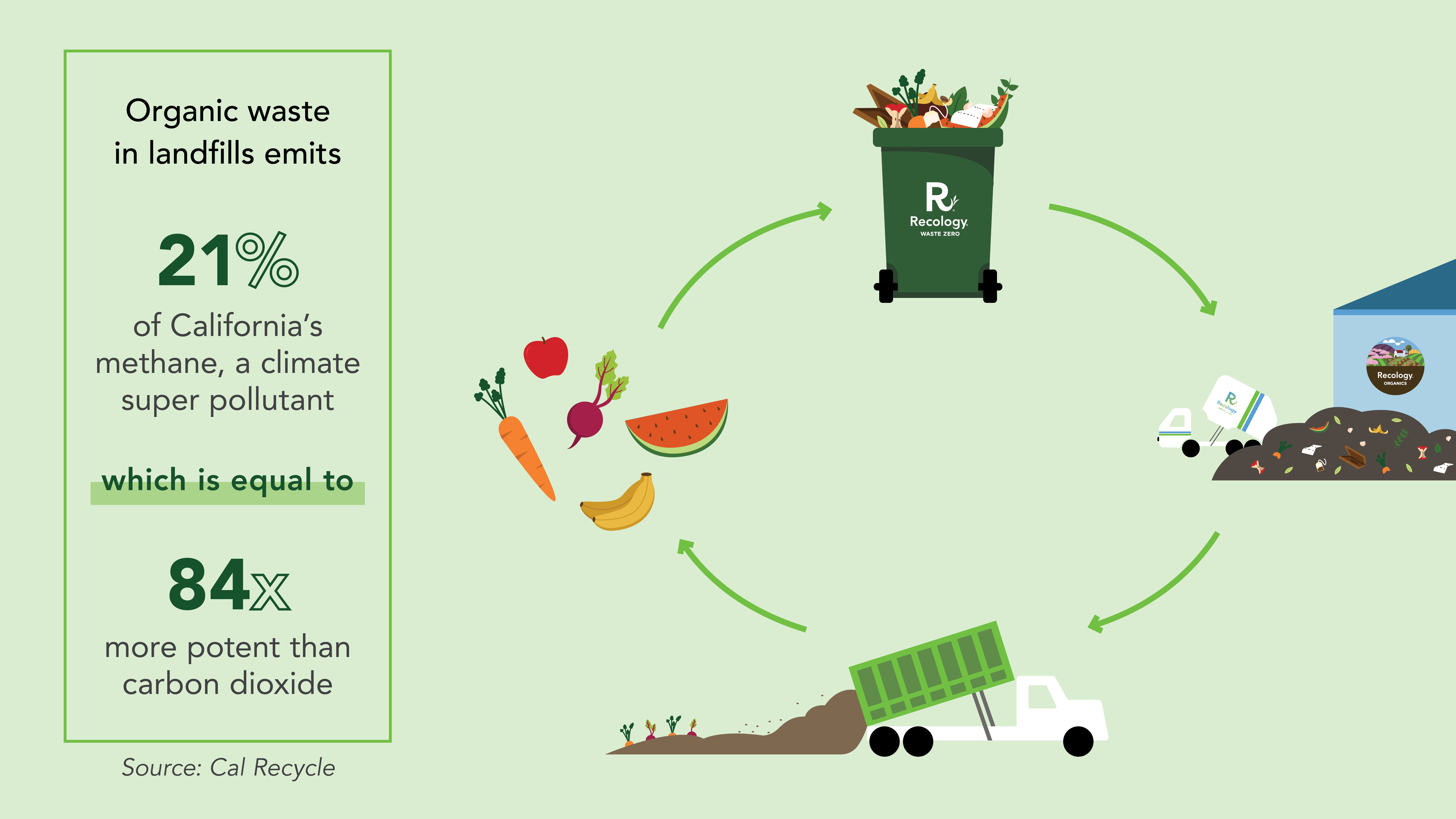This promotional image for recycling features a light green background and a central diagram illustrating the recycling process in a circular flow. Starting at the top, a green recycling bin labeled "Recology" is filled with various recyclable items. Following the arrow from the bin, we see a truck collecting the organic waste. The next step depicts a dump truck distributing compost soil over a garden, symbolizing the beneficial reuse of organic waste. The cycle continues with an arrow pointing to a variety of fruits and vegetables—banana, watermelon, apple, carrot, and beets—highlighting the end result of the composting process. The diagram completes the circle by returning to the recycling bin, reinforcing the sustainable loop of recycling organic materials into fertile soil and fresh produce. On the left side of the image, in bold black font, a critical message reads: "Organic waste in landfills emits 21% of California's methane, a climate super pollutant, which is 84 times more potent than carbon dioxide. Source: CalRecycle." This detailed visual and textual narrative effectively promotes recycling and raises environmental awareness.